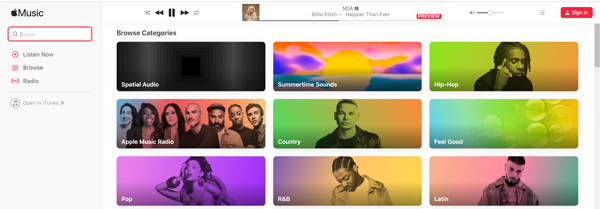This is a detailed screenshot of the Apple Music browser interface. On the left sidebar, there are options such as "Listen Now," "Browse," "Radio," and "Open in iTunes," along with a search bar for easy navigation. The central content area highlights the "Browse" category section. 

On the top-right section, there's a red "Sign In" button. Just below it, a "Now Playing" section displays the song "Noah" by Billie Eilish from the album "Happier Than Ever," accompanied by the album cover.

The main "Browse" area prominently features nine distinct categories arranged in a three-by-three grid. Each category is visually vibrant, with some sporting neon bright colors while others display artist photographs treated with neon bright filters. The categories are as follows:

1. **Spatial Audio**: Presented with a minimalistic blank screen.
2. **Apple Music Radio**: Features a diverse array of artist thumbnails with a blue-to-orange gradient background.
3. **Pop**: Showcases a female musical artist with a purple filter set against a white background.
4. **Summertime Sounds**
5. **Country**
6. **R&B**
7. **Hip-Hop**
8. **Feel-Good**
9. **Latin**

Each category is uniquely designed, providing a visually engaging way to explore different genres and featured content on Apple Music.